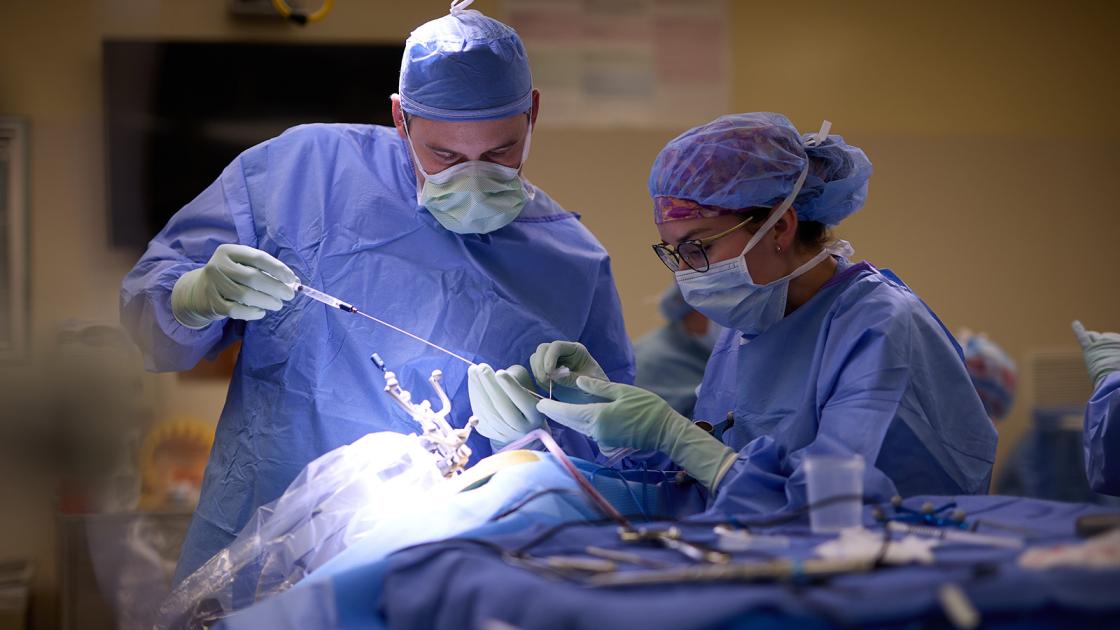The image features a meticulously arranged scene in a hospital operating room, showcasing two medical professionals—presumably a doctor and a nurse—engaged in a surgical procedure. On the left, a tall man in blue scrubs, a blue surgical cap, and a light blue mask is holding a long syringe with both hands. On the right, a woman, identifiable by her round, black-rimmed glasses, is assisting him by holding a small needle close to the syringe's tip. She wears a blue gown, white latex gloves, a pink handkerchief tied around her hair, and a blue hairnet over it. Both are focused on something off-frame, indicating a possible surgical site not visible in the image. A surgical table laden with numerous metallic tools and instruments is positioned at the bottom of the frame. The background reveals additional medical staff, also clad in blue scrubs, gloves, and masks, against walls painted a muted beige, completing the clinical and sterile ambiance of the room.